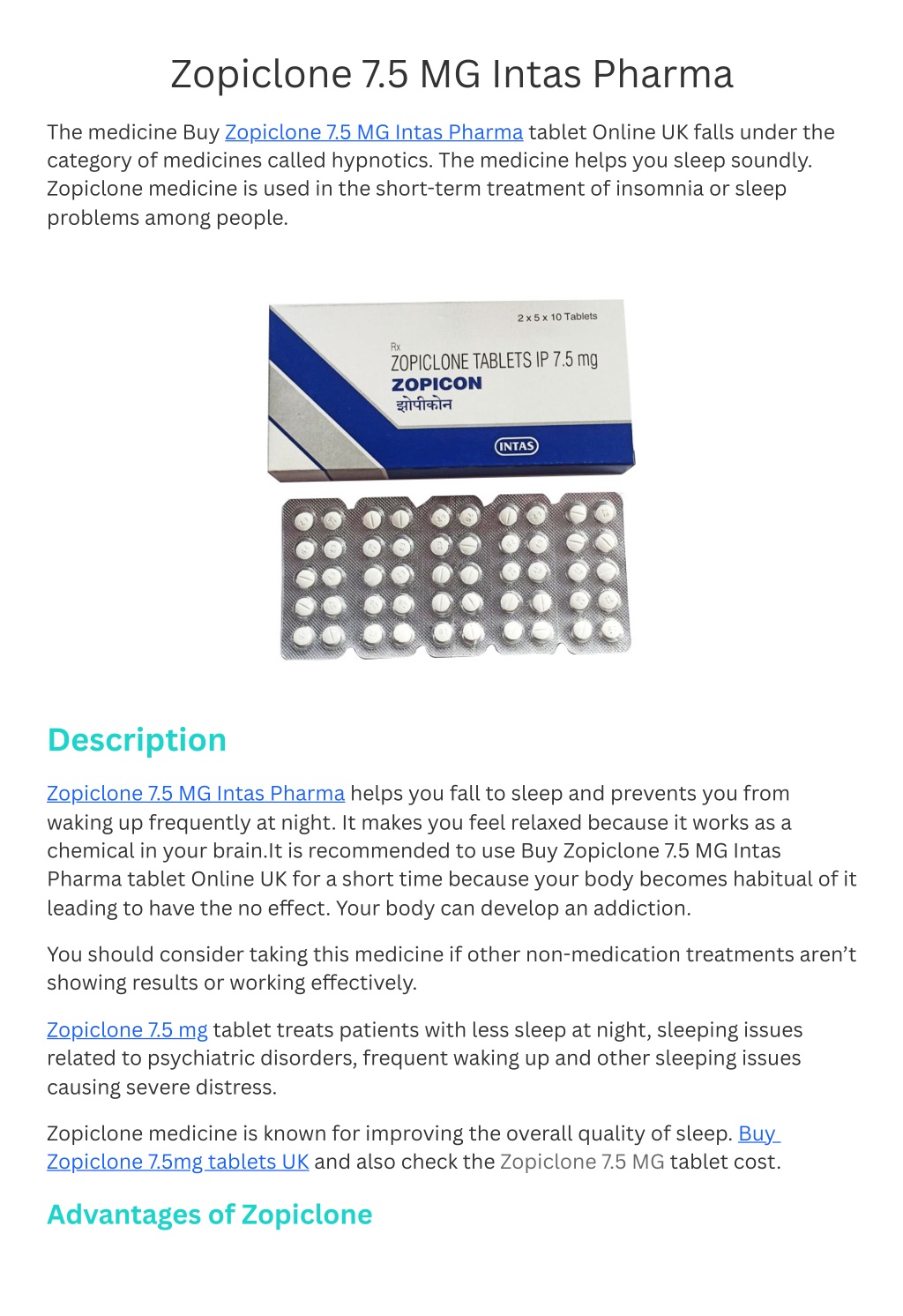The image displays a detailed description of Cyproclone tablets, specifically Cyproclone 7.5 mg by Instas Pharma. At the top of the image, bold text highlights "Cyproclone 7.5 mg - Instas Pharma." This medicine, available online in the UK, belongs to the category of hypnotics, aiding users in achieving sound sleep. It is primarily used for the short-term treatment of insomnia or other sleep-related issues.

Below this heading, there's a box in white, blue, and gray with the text "Rx Cyproclone Tablets IP 7.5 mg" followed by the brand name Cyproclone. The box includes Hindi script underneath, and visible in the image are the white, round tablets packaged in blisters.

Further down, the description elaborates that Cyproclone 7.5 mg from Instas Pharma helps users fall asleep faster and reduces frequent awakenings during the night. It creates a relaxing, soothing effect by acting on chemicals in the brain. However, it is recommended for short-term use to prevent the risk of habituation and potential addiction, as prolonged use might render it ineffective.

The text advises that Cyproclone should be considered when other non-medication treatments have failed to produce satisfactory results. It is beneficial for patients experiencing insomnia, sleep issues related to psychiatric disorders, and other conditions causing significant distress. The medicine is highly regarded for its ability to improve overall sleep quality.

Additionally, there is information on the advantages of using Cyproclone 7.5 mg tablets, including a focus on the cost-efficiency of the medicine. This part of the description is highlighted in a greenish-teal color.